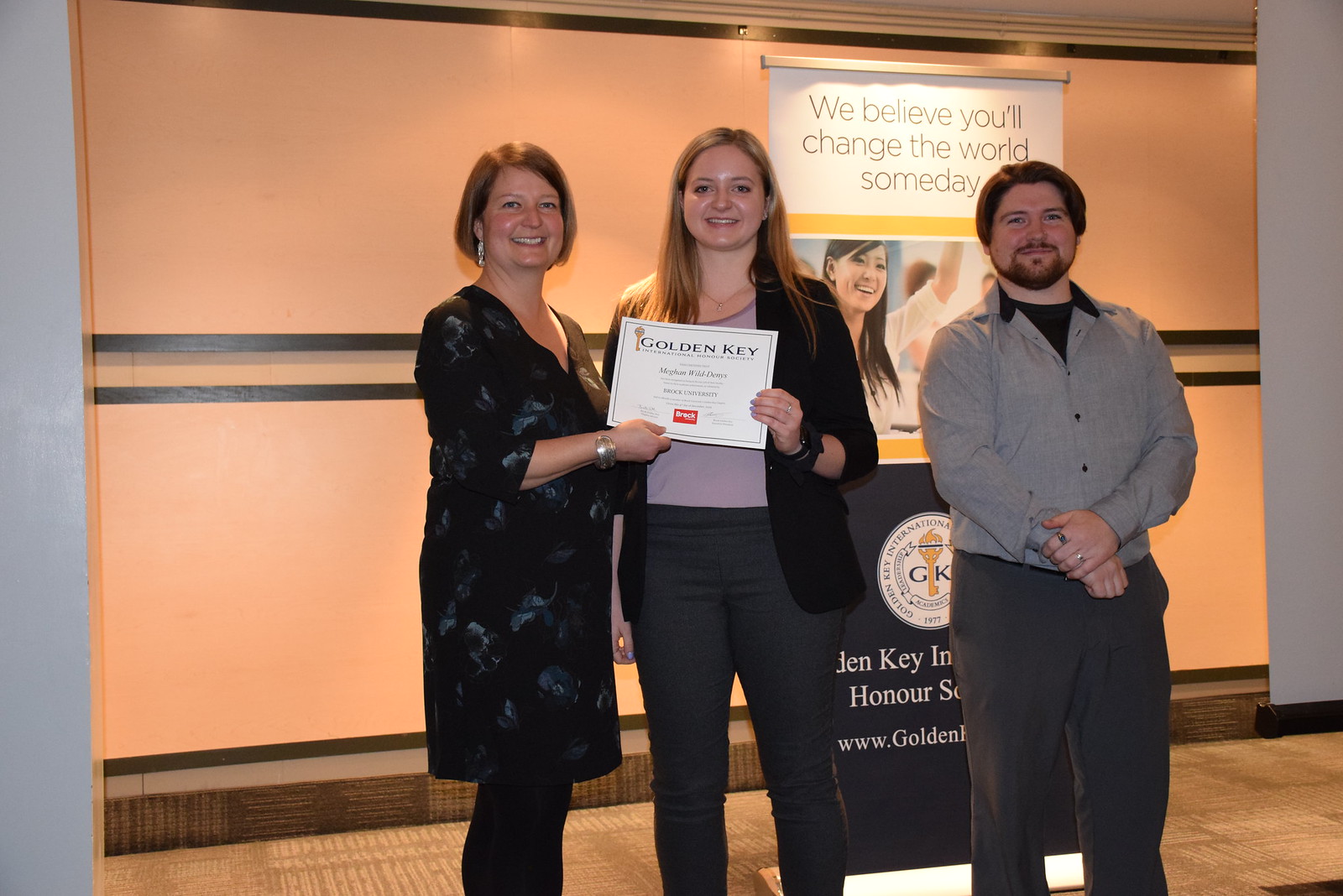The photograph captures three individuals posing in front of a step-and-repeat banner for the Golden Key International Honor Society, which reads at the top, "We believe you'll change the world someday." The scene is partially obscured but features text and logos related to the organization.

From left to right, the first person is a woman in her 40s, wearing tight black pants, a black dress adorned with a gray floral pattern, and silver dangling earrings. She is in the process of handing a white certificate with the text "Golden Key" to a younger woman in her 20s, who is at the center of the image. This younger woman, possibly a newly admitted Honor Society member, is dressed in tight gray pants, a purple scoop-neck blouse, and a black coat, and she holds the certificate with a proud demeanor.

To their right stands a man with a beard and mustache, dressed in gray pants and a light gray long-sleeve shirt with the top two buttons undone, revealing a black T-shirt underneath. His hands are clasped in front of him. The setting against the prominent banner, featuring motivational words and the society's logo, highlights the significance of the moment and the achievements being celebrated.